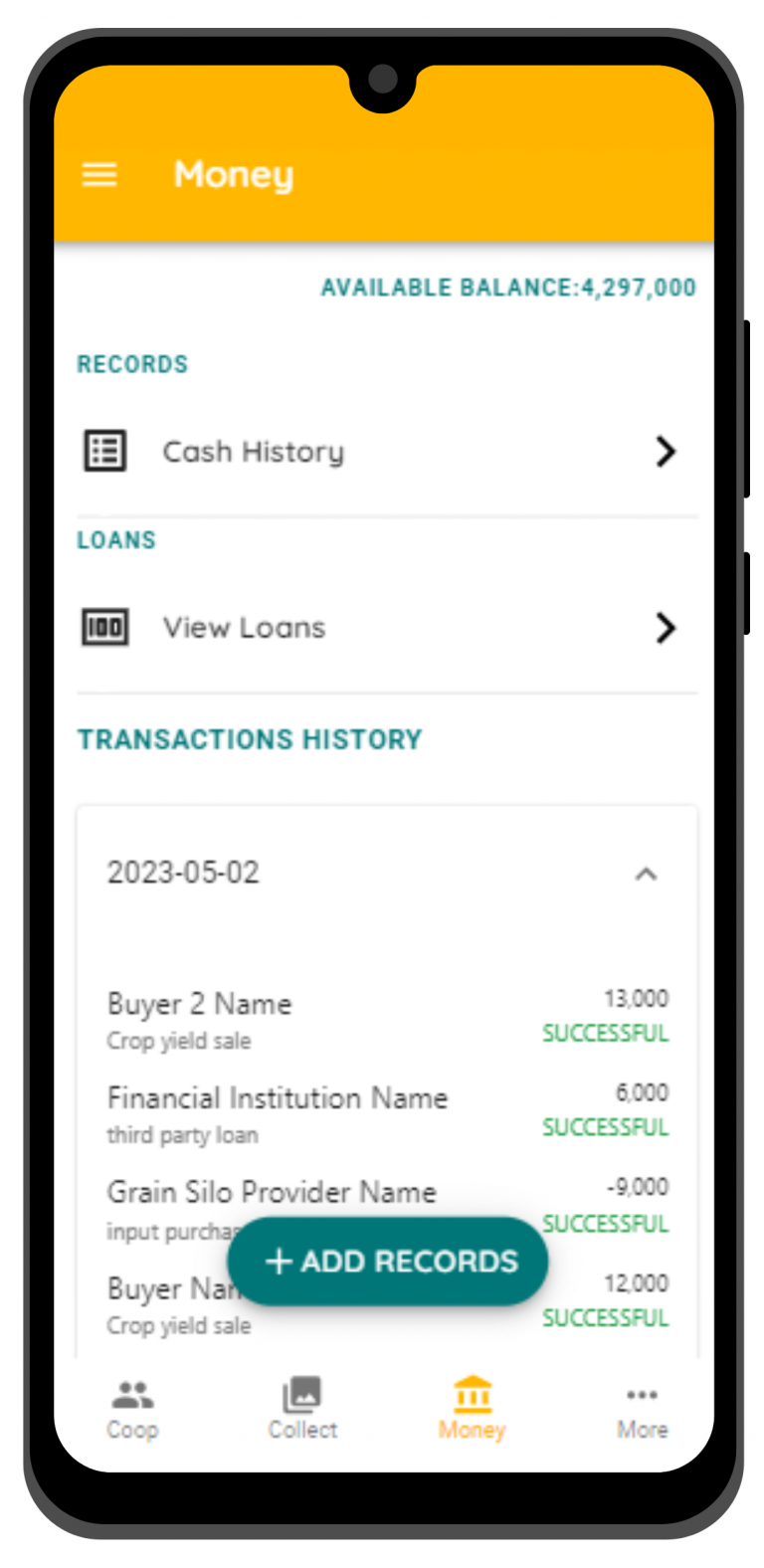A screenshot of a cell phone interface is displayed, bordered by a black outline mimicking the phone's edge. The top section showcases a prominent orange rectangle. Within this section, three horizontal white lines, representing a menu icon, are positioned on the left. Next to them on the right, the word "Money" is displayed in white text.

Beneath this, the background turns white. In the upper right corner, green text, capitalized, reads "AVAILABLE BALANCE" with a figure of "4,297,000" positioned directly below. 

Proceeding downwards, two lines below on the left, green capitalized text reads "RECORDS". 

Further below, a square encased in bold black outlines appears, filled with horizontal black lines, indicating a list or table. Adjacent to this on the right, the text "Cash History" is written, with a black right-pointing arrow, resembling a sideways "V", at the line's far end.

Continuing down, green capitalized text "LOANS" is visible. Another square follows, containing some black text inside. To the right of this square, "View Loans" is displayed along with a similar right-pointing arrow.

Further down, green capitalized text "TRANSACTIONS HISTORY" is shown. This is accompanied by a light gray outlined square. At the square's upper left corner, in gray text, the date "2023-05-02" is indicated. On the right side of this line, an upward-pointing arrow is present. Below these elements, a list of transactions is displayed with the transaction details on the left and corresponding dollar amounts on the right.